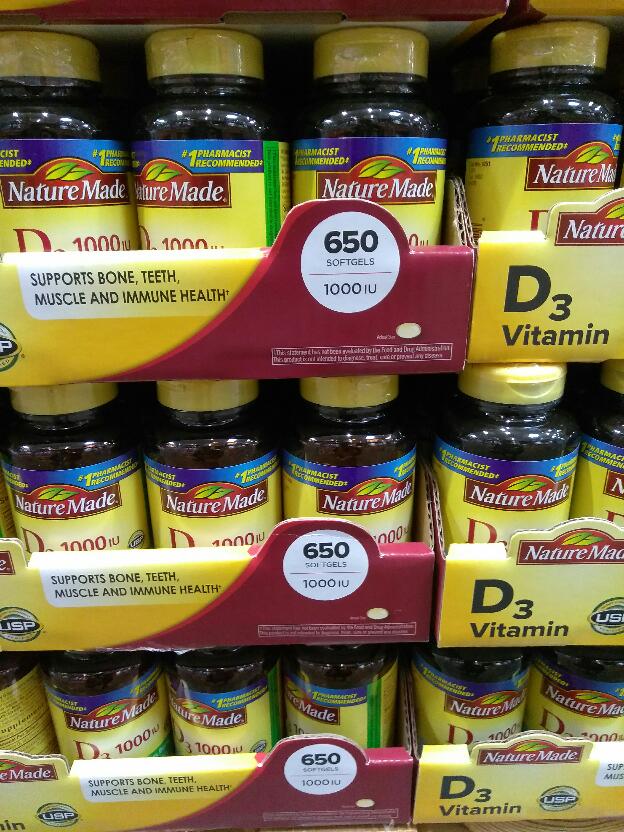This photograph captures an organized display of Nature Made vitamin packaging, typically seen in retail environments like grocery stores or big-box retailers, such as Costco. The vitamins are neatly stacked inside open-top cardboard boxes, engineered for both visibility and accessibility. Each box features a prominent design element: a bold red stripe adorned with a white circle that declares "650 soft gels" followed by "1000 IU." To the left of this circle, text highlights the health benefits of these vitamins, specifically noting that they support bone, teeth, muscle, and immune health. The arrangement and detailed labeling make it easy for shoppers to identify product benefits at a glance.